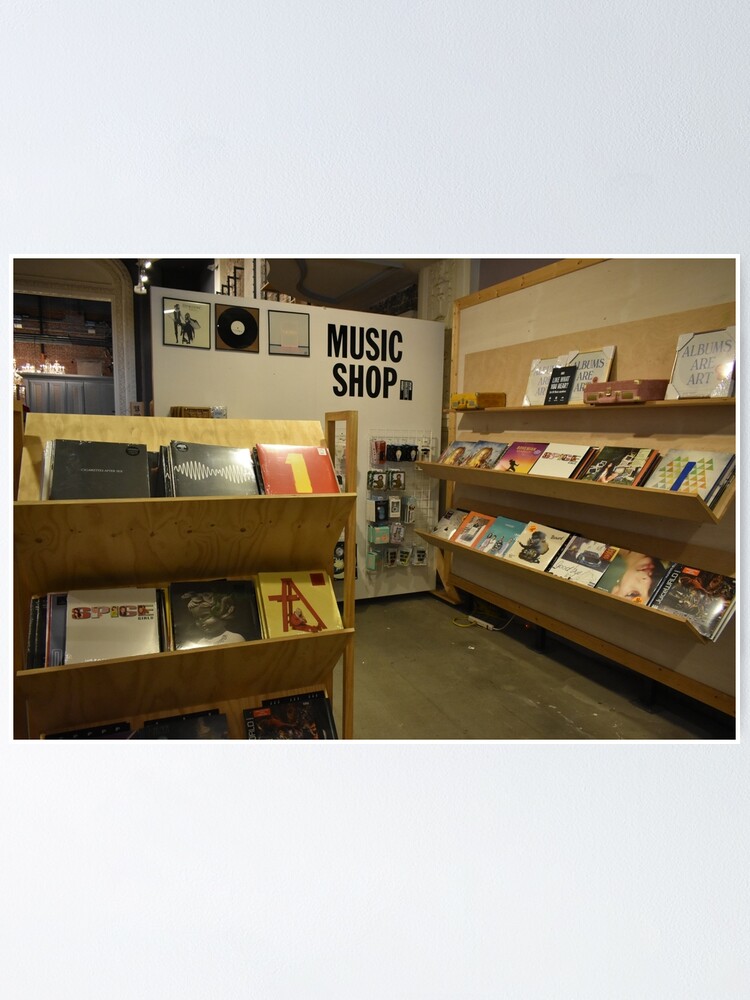The photograph captures the interior of a vintage record store featuring wooden floors that add a warm, welcoming touch. Dominating the left-hand side of the image, there are multiple shelves filled with albums and records, extending from the front to the middle of the scene. On the right, a wall runs into the depth of the picture, housing three angled shelves that provide easier access to the records displayed on them. Above these shelves is a collection of framed wall art, including one frame that declares "Albums are Art."

Further into the background, another wall painted white is prominently marked with the sign "Music Shop" in blue. Adjacent to the sign, several records are thoughtfully hung, enhancing the store’s nostalgic atmosphere. Below the sign and against the back wall, there is a rack that appears to hold various brochures or small items for sale, though the specifics are indistinct. Additional noteworthy elements include music players and possible A-tracks on the upper shelves, while another set of albums stands upright in the middle of the shop, inviting customers to browse through their selection.